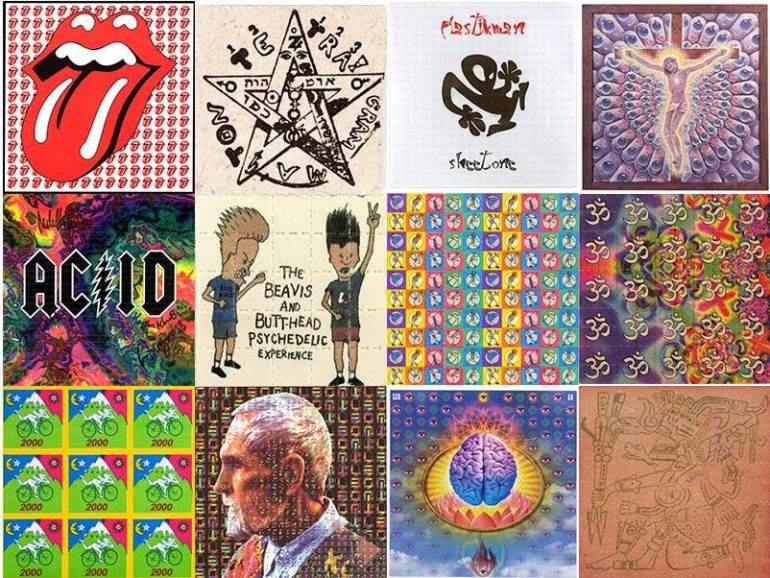This image is a detailed collage of 12 equally sized squares arranged in 4 rows and 3 columns, each featuring distinct patterns and pictures. On the top left square is a depiction of red lips with the tongue sticking out, reminiscent of the famous Rolling Stones logo. Adjacent to it is a star shape with some lettering. To its right is a Martian-like figure labeled “Plastic Man” in red letters, with "plastic" spelled with a 'K'. Beneath this figure, in obscure black letters, is the phrase "Skeet One." The top right square portrays Christ on the cross, against a peculiar background featuring various formations or possibly a pattern of eyeballs.

The second row includes a square displaying the word “ACID” designed to mimic the AC/DC band logo, followed by an image of Beavis and Butthead with the text “The Beavis and Butthead Psychedelic Experience.” There are also tiles featuring patterns of various colors such as purple, yellow, red, and green, interspersed among other images.

The collage continues with a mixture of visual elements and symbols across the remaining squares, including some hard-to-identify figures and images. These include a side profile of a person with short white hair and a white beard or goatee, a crescent moon, and a depiction of purple and blue brains within an oval, potentially surrounded by fire and mountains. There are also intricate line drawings of creatures and additional symbols, contributing to the composite’s psychedelic and eclectic nature.